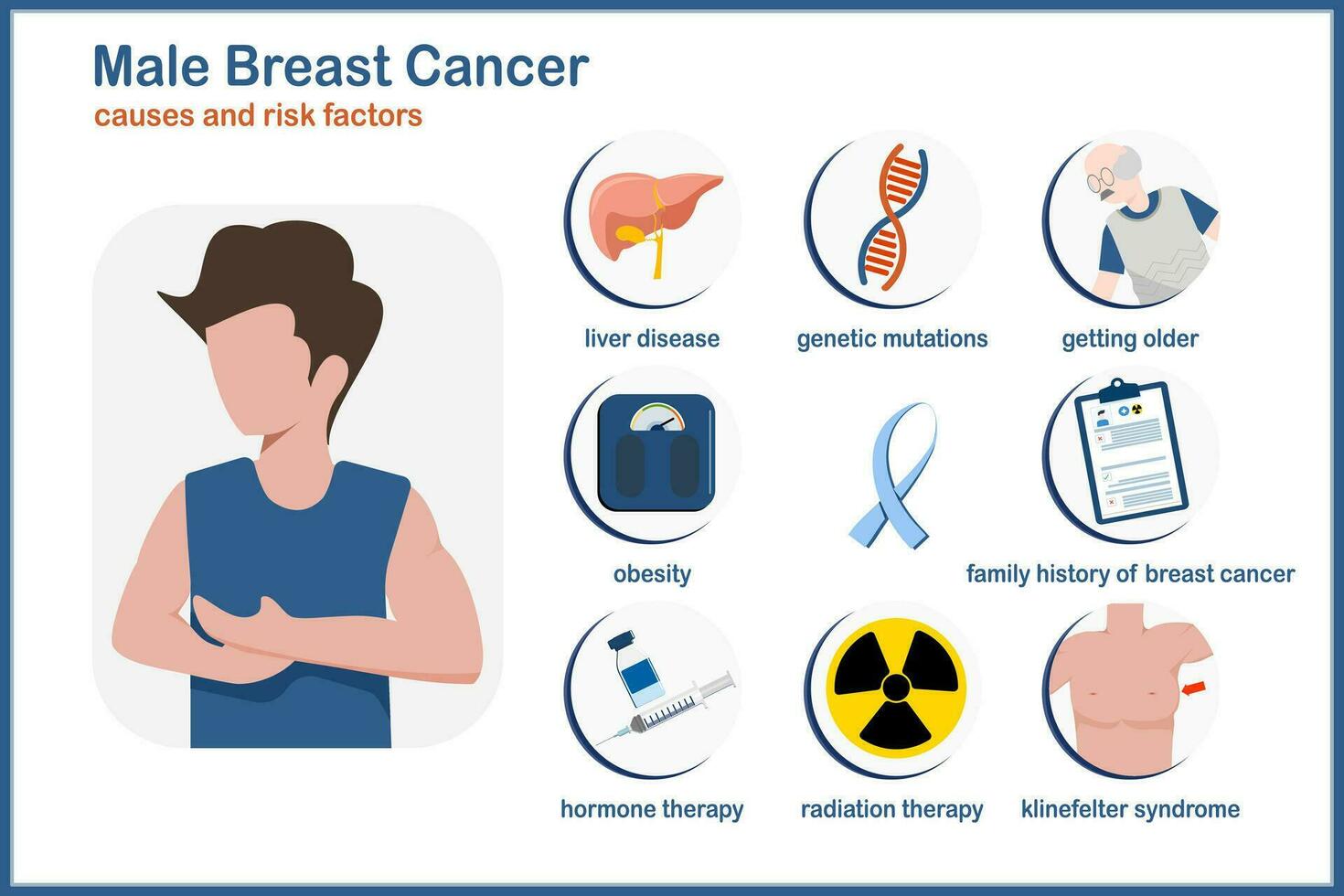The information graphic is centered on "Male Breast Cancer Causes and Risk Factors" and features a blend of visual elements to convey its message. On the left, there's a rectangular image of a faceless male figure with brown hair, wearing a blue tank top, and touching his chest. To the right, the graphic is organized into a grid of nine circles, each with vector art visuals relating to different risk factors.

In the first row, the circles depict a liver labeled "Liver Disease," a DNA sequence labeled "Genetic Mutations," and an elderly bald man labeled "Getting Older." The second row includes a scale labeled "Obesity," a blue ribbon symbol, and a clipboard labeled "Family History of Breast Cancer." The bottom row displays a vial and needle labeled "Hormone Therapy," a radiation symbol labeled "Radiation Therapy," and a torso labeled "Klinefelter Syndrome."

This well-designed, detailed chart succinctly outlines key causes and risk factors of male breast cancer with associated visuals to enhance understanding. It appears best suited for educational settings, given its clear and informative presentation style.